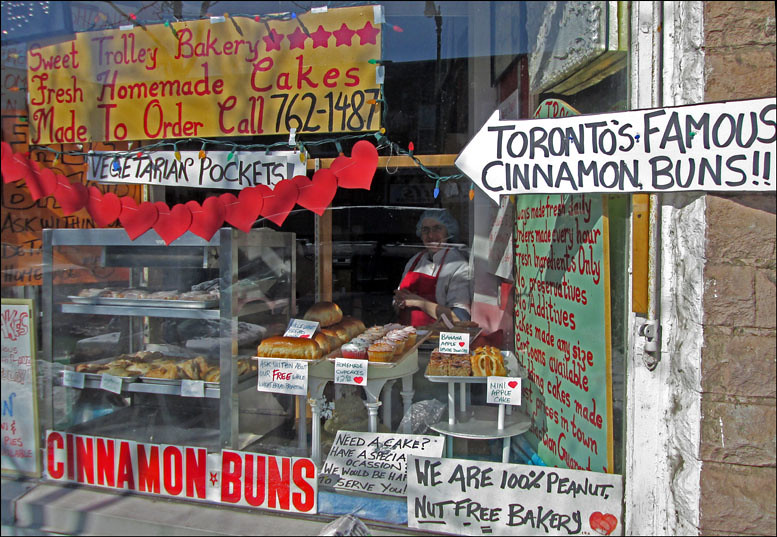The photograph captures the charming storefront of Sweet Trolley Bakery, taken from outside through a large glass window. Prominent signage in bright red text on a yellow background at the top of the window announces, "Sweet Trolley Bakery. Fresh Homemade Cakes Made to Order. Call 762-1487." Just below, a white sign with black text lists, "Vegetarian Pockets." 

An arrow on the exterior brown brick wall points towards the bakery, boldly proclaiming, "Toronto's Famous Cinnamon Buns." The window itself displays several signs, including large red lettering at the bottom that reads, "Cinnamon Buns," and another sign confirming it is a "100% Peanut Nut-Free Bakery," accentuated with a heart. Additionally, a festive banner of red hearts is strung across the window, complemented by a series of unlit Christmas lights.

Inside, a cheerful woman wearing a red apron over a white shirt and a hairnet smiles directly at the camera. The display case in front of her is filled with an enticing assortment of baked goods, including cupcakes, éclairs, muffins, and perhaps mini apple cakes. The sunny day outside bathes the entire scene in natural light, highlighting the delightful and welcoming atmosphere of the bakery.